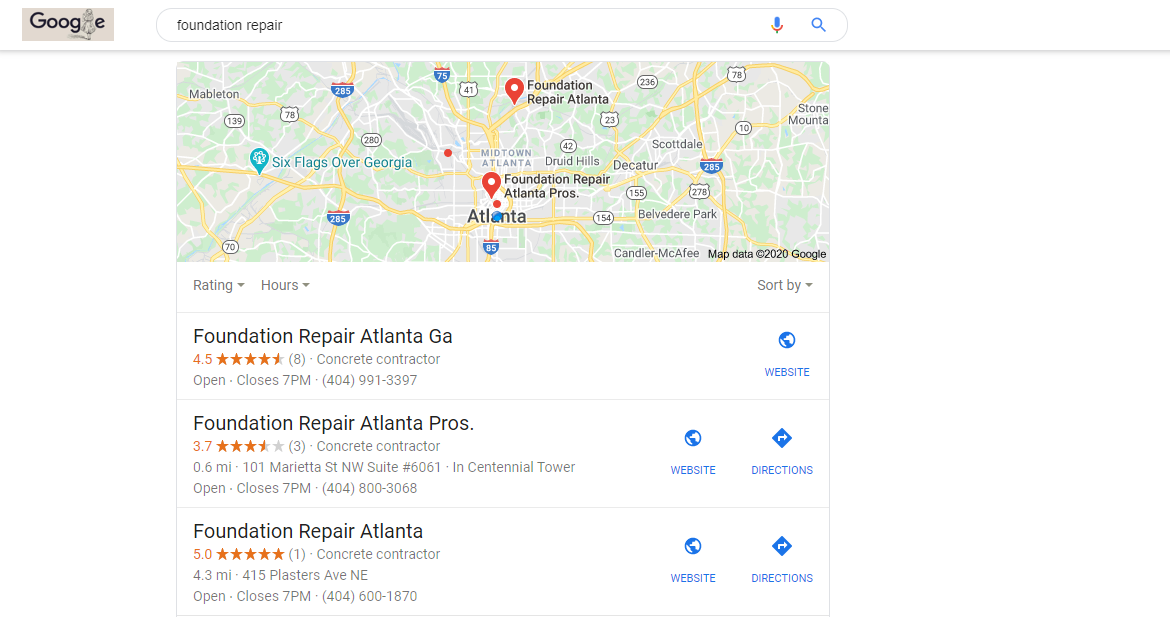This is a screenshot displaying the top portion of a Google search results page for the term "foundation repair." At the top of the page, the search bar clearly shows the query "foundation repair." Below the search bar, a segment of the Google Maps interface is visible, highlighting the greater Atlanta area. Within this map segment, two red location pins mark specific foundation repair service providers: one situated centrally at the top of the map and the other positioned closer to downtown Atlanta.

The map header is followed by three text-based search results. The first result appears under the name "Foundation Repair," specifically serving the Atlanta, Georgia area. The second result, similarly labeled "Foundation Repair Atlanta, Georgia," indicates a broader service range within the region. The third result is listed as "Atlanta Pros," offering specialized foundation repair services within the city. The detailed display of these search results provides a concise overview of available foundation repair options in the greater Atlanta area.